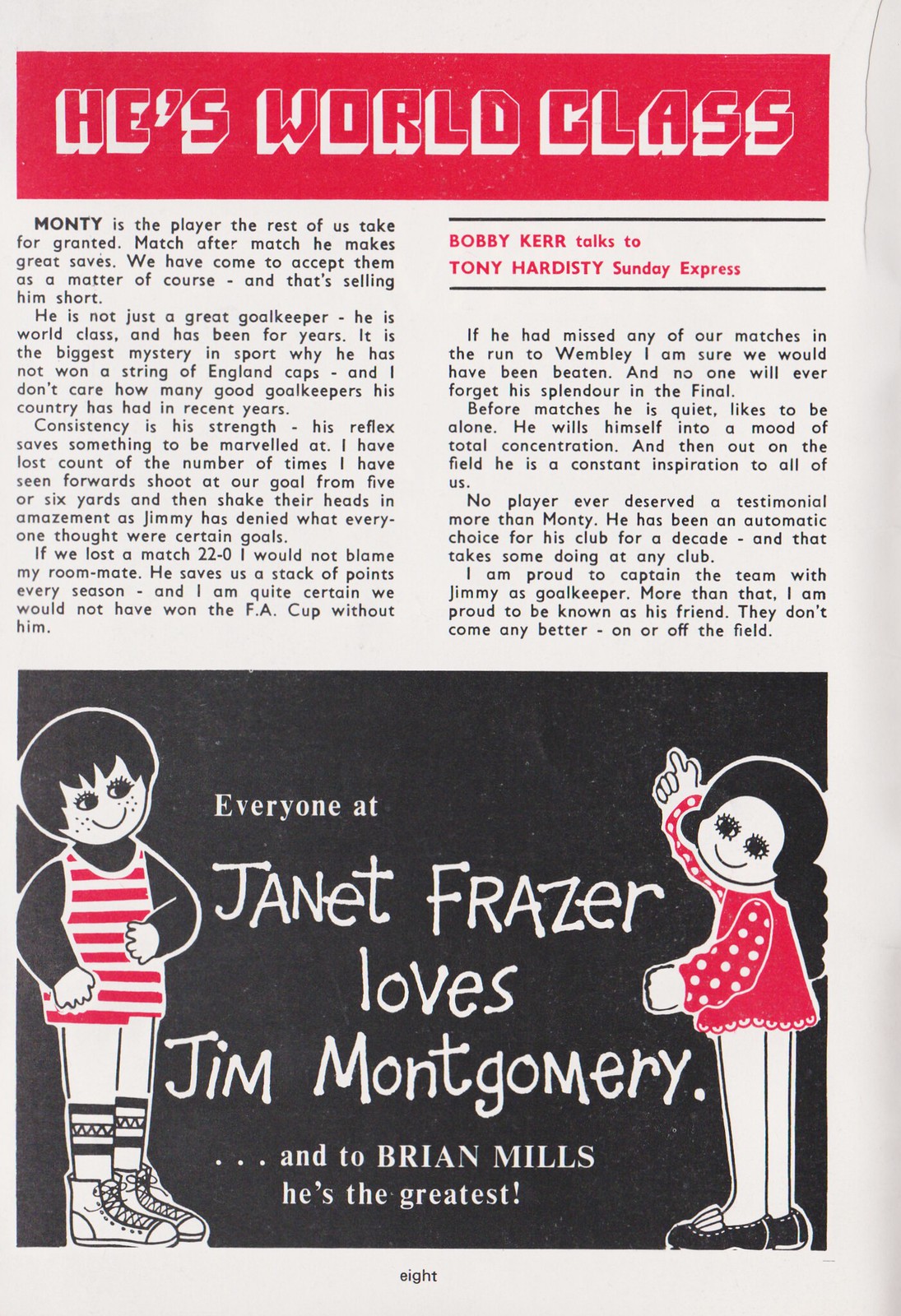This image, appearing on page 8 of a Booker magazine, features a light gray background topped by a red rectangular box with red and white shadowed letters proclaiming "He's World Class." The article is focused on the soccer goalie, Jim Montgomery, often referred to as "Monty." The headline, "Bobby Kerr talks to Tony Hardesty, Sunday Express," is prominently displayed. The first part of the article reads, "Monty is the player the rest of us take for granted. Match after match, he makes great saves. We have come to accept them as a matter of course, and that's selling him short."

At the bottom of the image, there is a drawing set against a black background featuring two animated characters. On the left, a boy with short black hair wears a long-sleeved shirt with red and white stripes and sneakers with long socks. On the right, a girl with long braided black hair wears a lacy red dress with white polka dots on the sleeves and black shoes. Between them, white text reads, "Everyone at Janet Frazier loves Jim Montgomery... and to Brian Mills, he's the greatest."